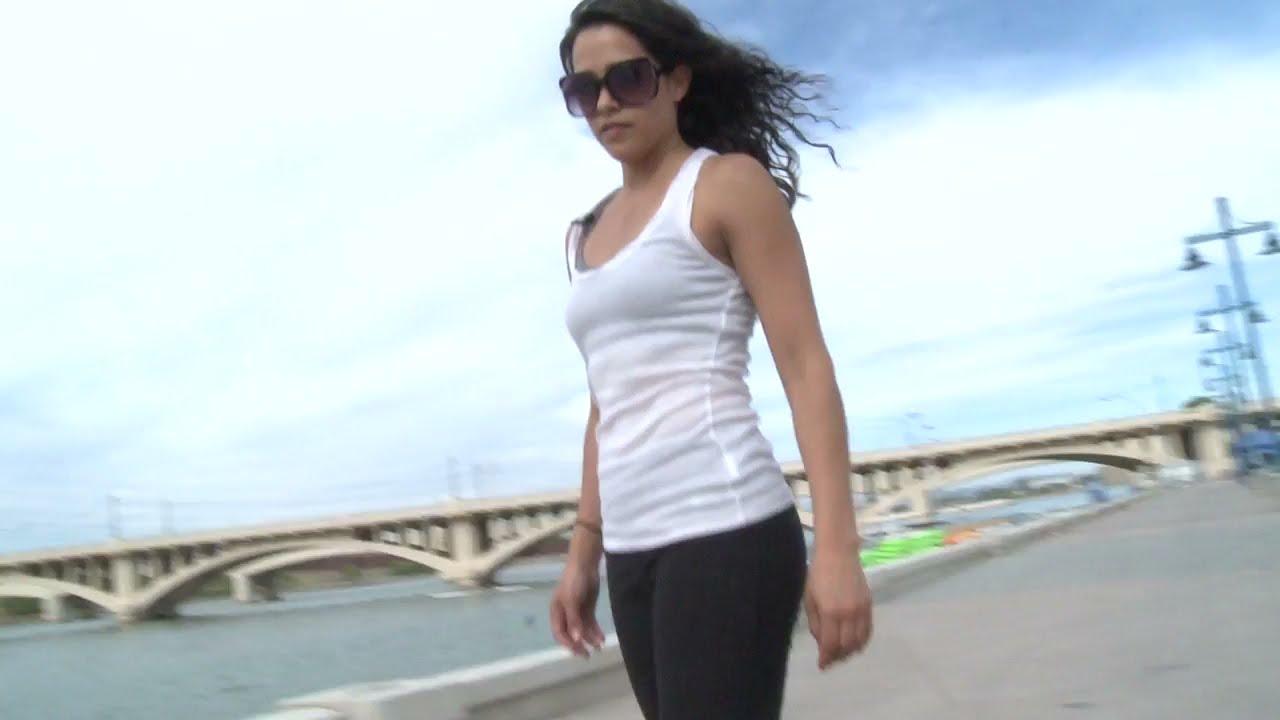The horizontal rectangular color photograph captures a unique perspective of a woman in her late 20s or early 30s in an outdoor park area. She is dressed in a white tank top, black capri athletic pants, and gray Nike shoes, holding hand weights down by her sides. The image emphasizes her standing in the grassy park next to a public walkway or track, with green lampposts and a couple of gray lanterns around her. In the far background, there's a modern, circular-fronted, ten-story glass building, giving the illusion that she is taller than the structure due to the camera angle. Additionally, a bridge, likely over a highway or river, spans the distance with trees and various park amenities like benches and trash cans visible. The overcast sky with many clouds adds a subdued tone to the scene as she appears poised to either take a step or begin her exercise routine amidst the well-lit, landscaped surroundings.